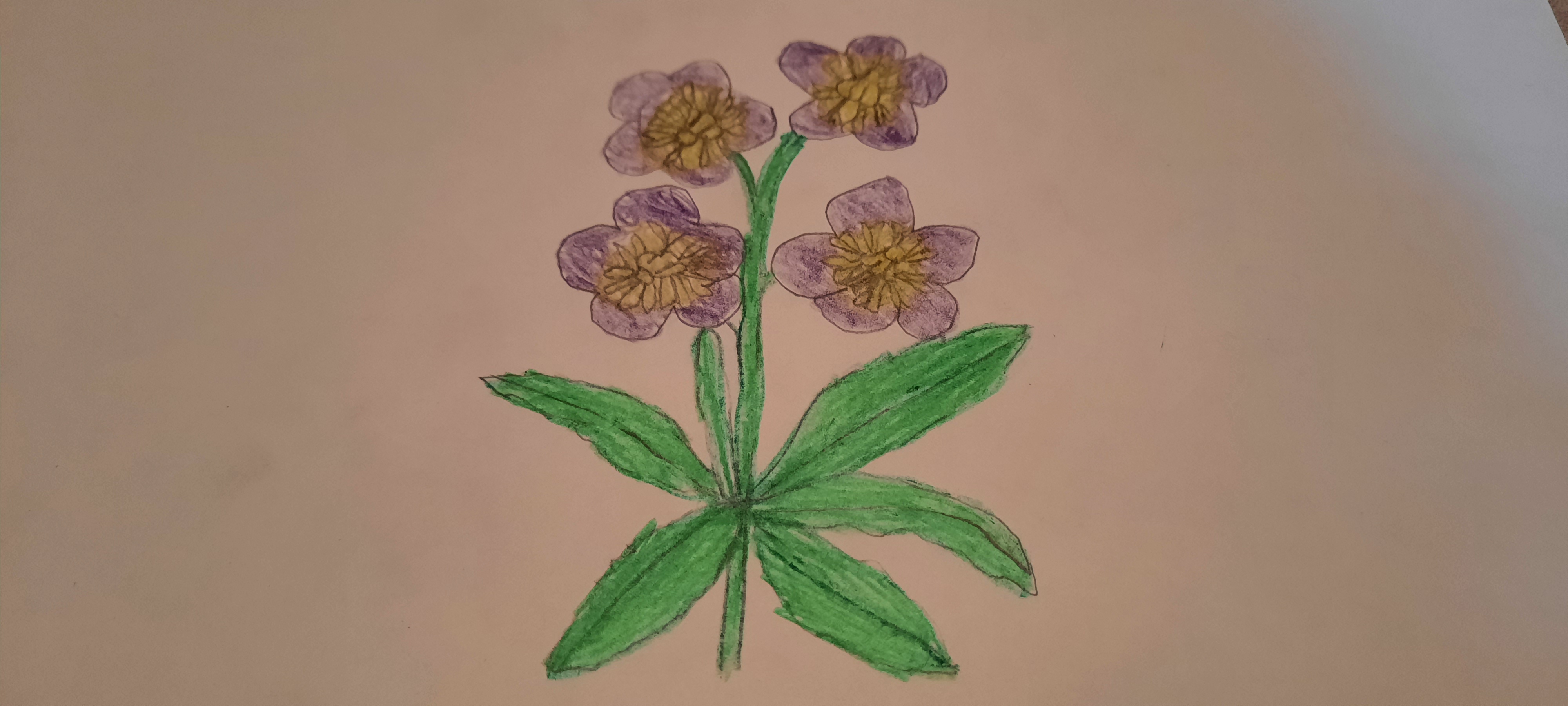The image depicts a child-like drawing crafted with colored pencils or crayons, featuring a flower with a bright green, long stalk on a landscape-oriented, blank white piece of paper. The flower's stem is outlined in black and extends vertically, branching out at the top to support four purple flowers, each distinguished by five petals and vivid yellow stamens at the center, resembling semi-oval pollinators. The arrangement consists of two flowers on the left and two on the right, with a secondary branch extending to the first left flower. Below the flowers, the stem bears six pointed, oval-shaped green leaves, three on each side, adding a balanced, vibrant touch to the whimsical botanical illustration.